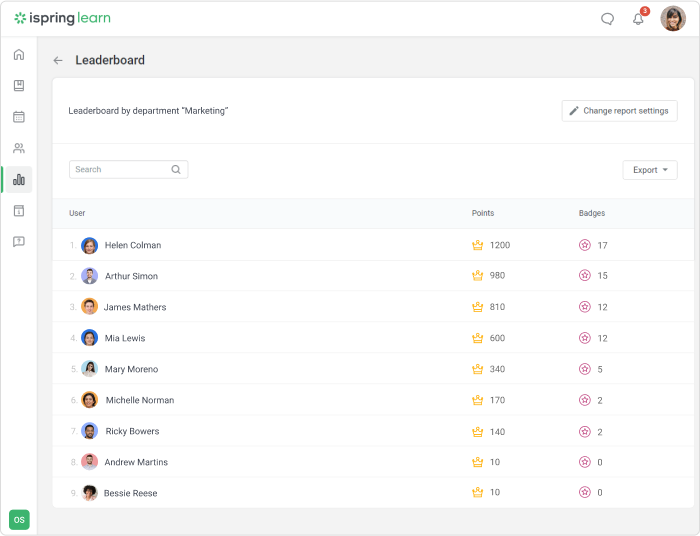The image showcases a digital interface of iSpring Learn, identifiable by the logo prominently displayed at the top. On the right corner, there's a profile picture of the user who has accessed this page. The interface is focused on a section for the marketing department within a company, displaying a leaderboard dedicated to the department's learning progress.

The leaderboard currently highlights nine users, each represented by a circular profile picture accompanied by their name. Starting from the top, Helen Coleman is ranked first with a remarkable 1,200 points, symbolized by a gold crown, and has earned 17 badges. Following her is Arthur Simon with 980 points and 15 badges, James Mathers with 810 points and 12 badges, and Mia Lewis with 600 points and 12 badges. Lower down the ranking, Mary Moreno holds fifth place with 340 points and 5 badges. The list continues down to Bessie Reese in ninth place with 10 points and no badges. Each user's position, points, and badges are clearly indicated next to their profile, emphasizing their learning achievements within the department.